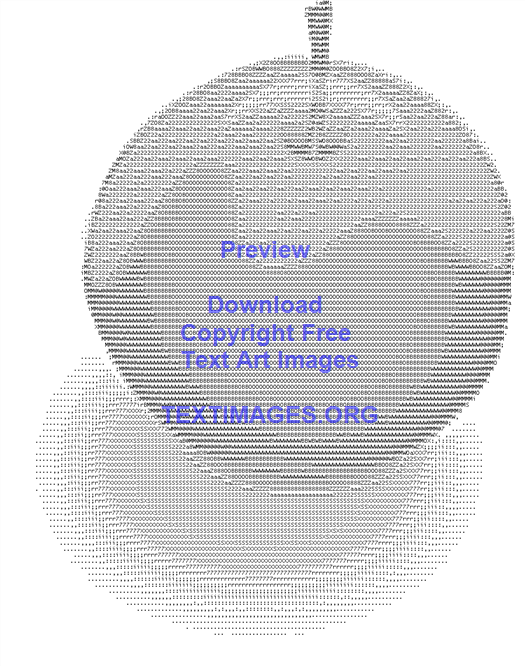The image, sourced from textimages.org, features a detailed text art rendering of an apple prominently set against a white background. The apple itself is intricately shaded using various text characters, including Rs, Xs, 2s, As, 0s, and carets, creating an impressive grayscale effect with light and dark gray tones. The text elements meticulously combine to depict not only the apple but also a subtle shadow beneath it, further enhancing the three-dimensional appearance. At the top of the apple, the phrases "Preview," "Download," "Copyright Free," "Text Art Images," and "TextImages.org" are displayed in legible light blue text. These lines serve to inform viewers of the image's source and availability, emphasizing that the art can be freely obtained from textimages.org. This cleverly composed piece demonstrates the creative potential of using text characters to form visually compelling images.